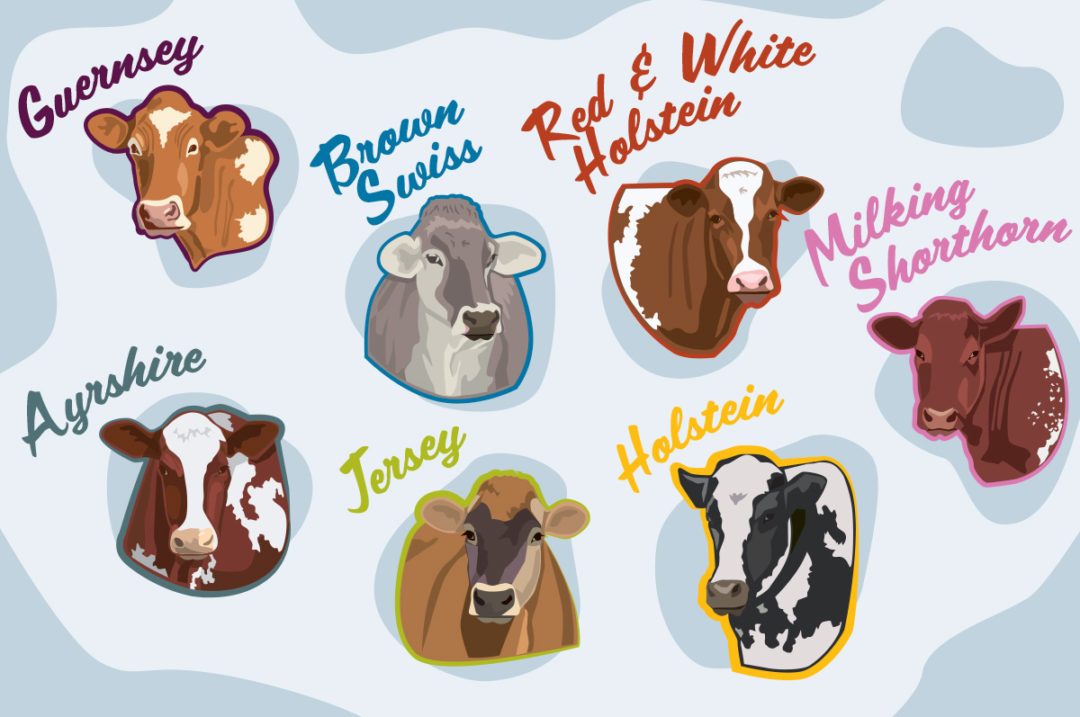This rectangular illustrated image features seven different cows, each depicted from the head and front shoulders, all looking directly at the viewer. They are set against a light gray background with darker gray circles. Each cow is uniquely colored and labeled with its corresponding breed in distinct colored cursive text. From left to right, the cows are: a brown cow with white spots labeled "Guernsey" in purple text; a gray cow with a brownish nose labeled "Brown Swiss" in blue text; a brown and white cow labeled "Red and White Holstein" in red text; a dark brown cow with small white spots labeled "Milking Shorthorn"; a classic black and white cow labeled "Holstein" in yellow text; a tan and gray cow labeled "Jersey," and a white and brown cow labeled "Ayrshire" in varied text colors.